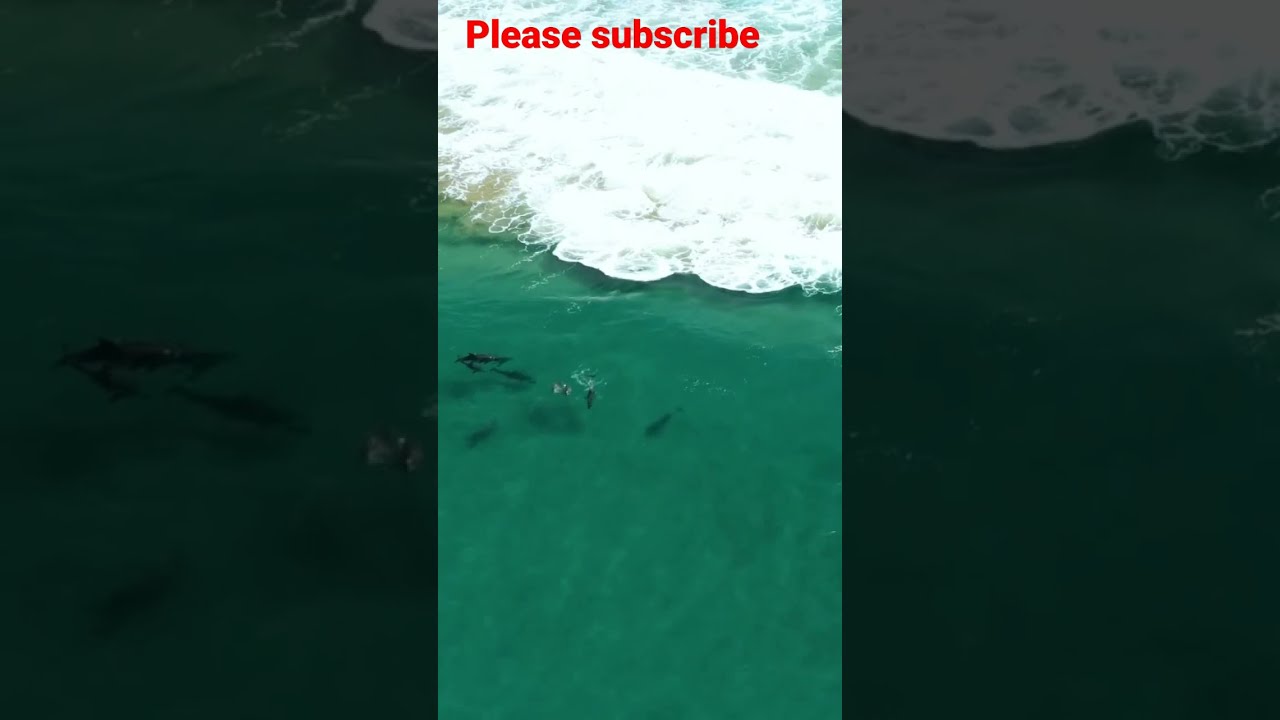This aerial photograph showcases a stunning ocean scene featuring remarkably clear, greenish-turquoise water. Prominently, a large wave, its white foam crests creating a striking backdrop, spans across the upper portion of the image. In the translucent water below, numerous fish are visible, particularly concentrated towards the center and left side. Approximately five to six fish are clearly swimming in the center, while larger fish, possibly sharks or dolphins, can be spotted to the left. The image conveys a fascinating marine snapshot, likely captured from a helicopter. At the top of the image, fairly well-centered, bold red text reads "Please Subscribe," indicating it might be from a video channel seeking subscriptions.